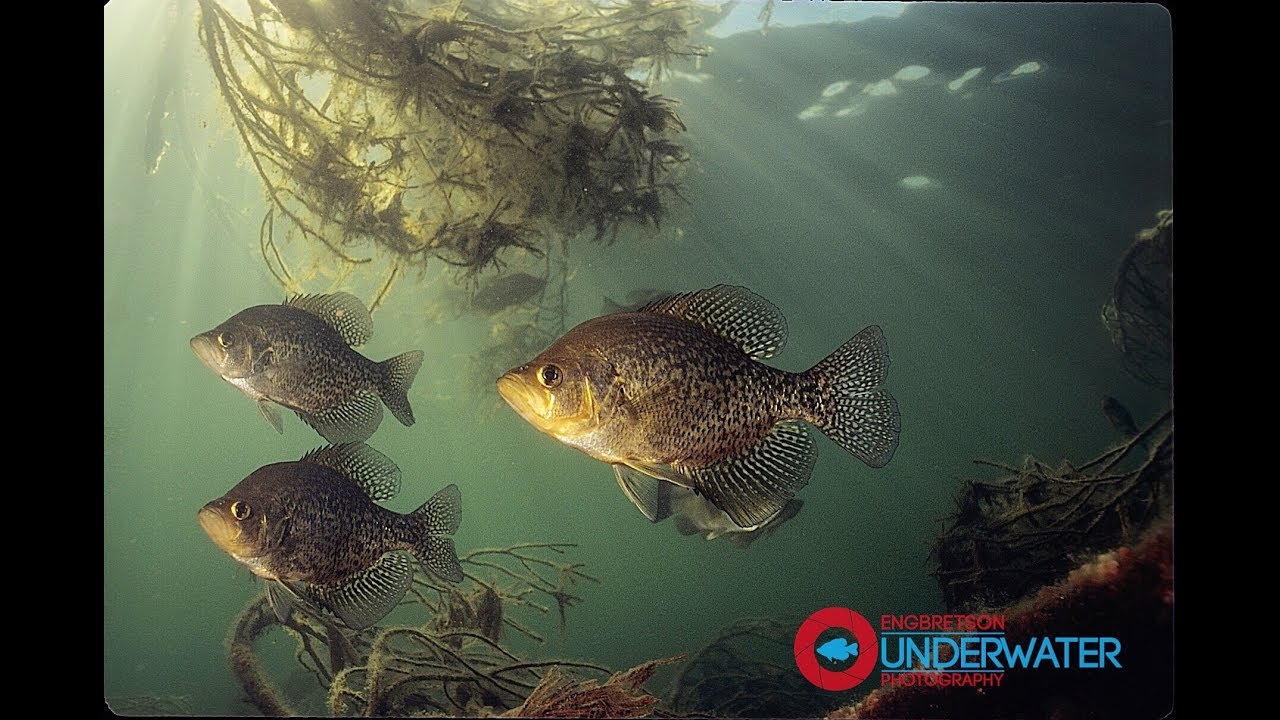This underwater photograph, possibly taken in a lake, showcases three fish as the central focus. In the foreground, two smaller spotted fish are positioned one above the other; both exhibit a mix of silver, black, and some hint of yellow around their mouths. The upper fish is primarily silver while the lower one has a distinct yellow patch beneath its mouth. Behind them, a larger fish of the same species also shows more pronounced yellow under its mouth, contributing a sense of depth to the image. 

All fish feature characteristic black spots and fins adorned with black and white polka dots. Above them, green seaweed floats, partially submerged, with sunlight piercing through the water, casting visible rays. At the bottom of the picture, more seaweed and algae are evident, further enriching the aquatic scenery. Finally, in the bottom right corner, the logo of Engbretsen Underwater Photography is visible, consisting of a blue fish silhouette within a red ring, with the text engraved in blue and red.